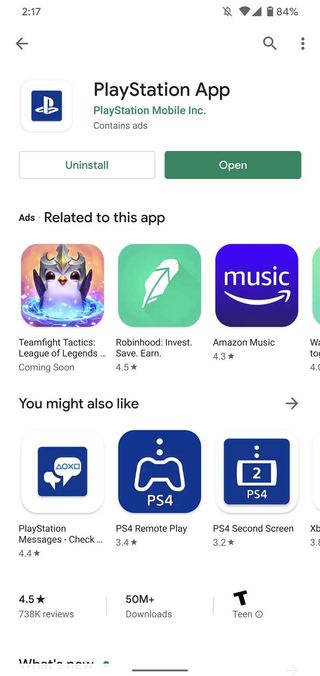A cell phone screenshot shows the screen at 2:17 (the absence of AM or PM is noted). The phone is in Do Not Disturb mode with notifications on, connected to Wi-Fi, and displaying a full cellular signal. The battery is at 84% charge. The interface includes a back button, a search bar, a search button, and a three-dot menu icon.

The main section features the PlayStation app, with its logo and developer name, PlayStation Mobile Incorporated, noting that it contains ads. There are options to uninstall or open the app. Below that, ads related to this app are displayed: "Team Fight Tactics," "League of Legends: Coming Soon," "RobinHood," and "Best Dave Earn," with ratings such as 4.5 stars. 

Further down, there is a "Music from Amazon" ad with a 4.3-star rating. The section titled "You Might Also Like" offers more suggestions with a right-arrow indicating additional options: "PlayStation Messages" (4.4 stars), "PS4 Remote Play" (3.4 stars), and "PS4 Second Screen" (3.2 stars).

The PlayStation app details further include a 4.5-star rating, based on 738,000 reviews, with over 50 million downloads, rated T for Teen, along with a brief section titled "What's New."